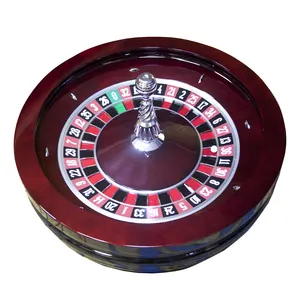The image displays a dazzlingly bright casino roulette wheel, set against a stark, plain white background. The wheel, which is round and cup-shaped, features a maroon-colored rim. At the center, there is a raised, dome-shaped section resembling the top of a king chess piece, adorned with a spiral silver metal piece capped at the summit. Surrounding this central elevation is a ring of alternating black and red numbered wedges, with a single green wedge that stands out. The numbers on the wedges include a black 26 and a red 3, among others, while the green wedge, marked with a '0', extends slightly beyond the inner circle to the outer edge. The overall brilliance and lack of background details create an almost blinding, glaring effect. This uniquely vibrant depiction captures the essence of a roulette wheel, a staple in many casinos.